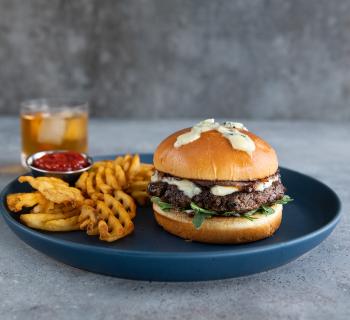This close-up image captures a delectable meal on a blue ceramic plate set against a light gray table with a darker gray wall in the background. The centerpiece is a juicy beef hamburger adorned with a toasted bun, arugula, grilled onions, and a dollop of aioli on both the top bun and patty. There's a layer of melted white cheese, and a light sprinkling of parsley adds a touch of elegance. To the side, a generous portion of waffle-cut French fries accompanies the burger, along with a small steel bowl — containing about a quarter to half a cup of ketchup. In the blurred background, an amber-colored beverage with ice, possibly iced tea, rests in a glass, suggesting a refreshing accompaniment to the meal. This setting indicates an upscale restaurant rather than a fast-food joint, promising a well-crafted dining experience.